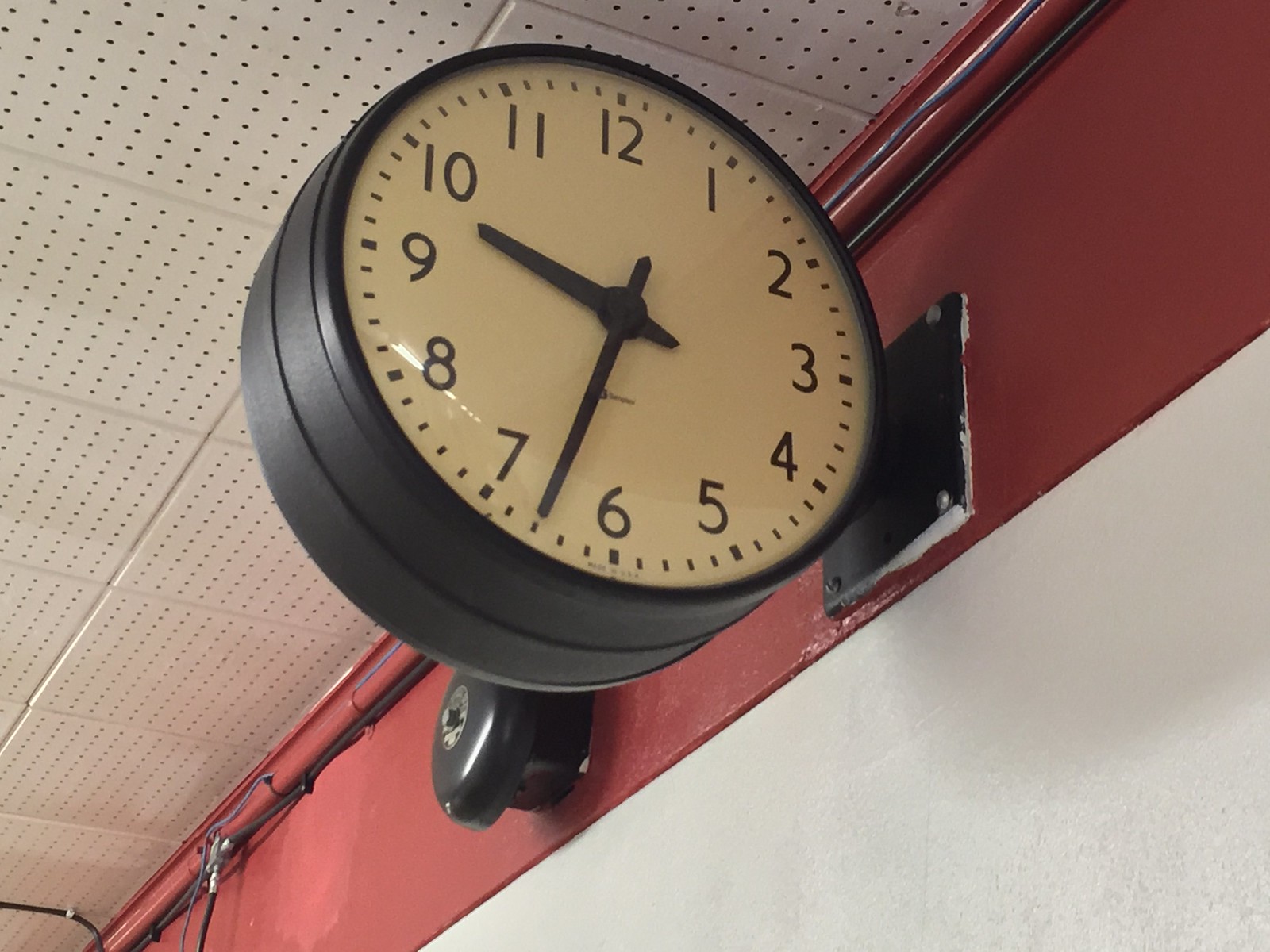The image features an old, classic analog clock mounted high on a white wall, near the ceiling. The clock has a black frame with a stark white face, showcasing black numerals from one to twelve. Both the hour and minute hands are black, and the clock lacks a second hand. The brand name on the clock face is illegible. Adjacent to the clock is a school bell, hinting at the setting being a school, where the bell likely rings loudly to signal class times. The clock appears to be electric, securely fastened to the wall with visible screws. The upper portion of the wall features red wainscoting, and the ceiling has a pattern of foam tiles that likely contribute to acoustic damping in the room. The photograph is remarkably clear, emphasizing the details of the clock and its surrounding environment.